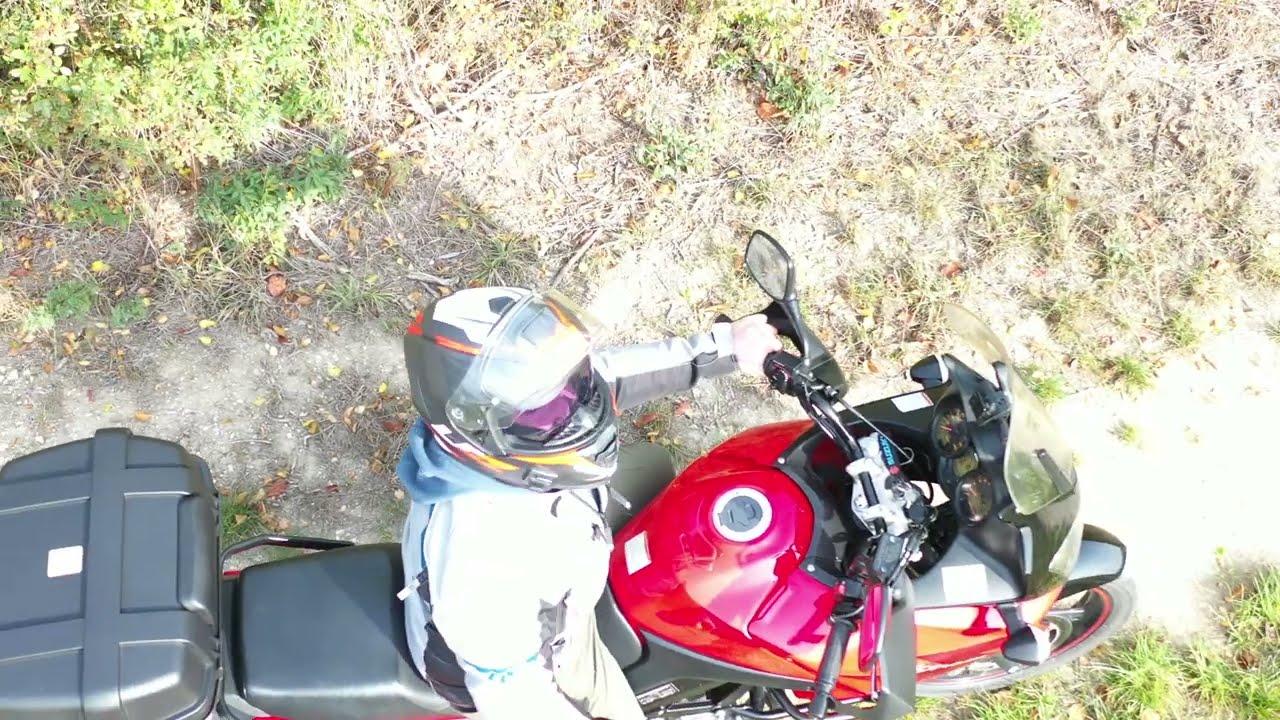Captured from an aerial perspective by a drone hovering just above, this detailed image showcases a man on a shiny, new, red BMW enduro-type motorcycle, designed for both on-road and off-road use. The rider, donning a gray helmet with the visor up and a white and black motorcycle riding jacket, is positioned on a dirt track surrounded by grass and fallen leaves, suggesting a rustic, natural environment. His one hand grips the handlebar while the other is on the throttle, indicating he has stopped, perhaps to take in the scenery. The motorcycle features a small windshield, an instrument cluster with a tachometer, speedometer, and fuel gauge, as well as a small trunk space mounted on racks behind the passenger seat. The intense lighting from the front adds a dramatic effect, enhancing the vibrant colors of the scene.